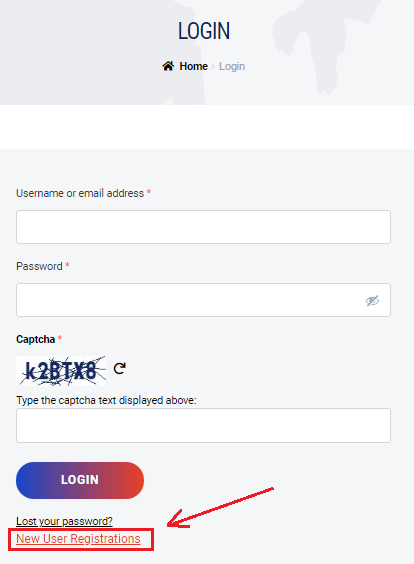The screenshot depicts a login page interface. At the top, the page title "Login" is prominently displayed alongside a home button, which features a house icon and is styled in bold black text. However, the login button at the top is grayed out, indicating it is currently inactive. 

Beneath this header, there is a gray box containing the input fields for logging in. These white input fields are clearly labeled, starting with "Username or Email Address", marked with a red asterisk to indicate that it is a required field. Below this is another input field for "Password," which is also required. Next to the password field, an eye icon (represented as a small cross) allows users to toggle the visibility of their password to see what they are typing.

Further down, there is a CAPTCHA verification section, a security measure to prevent automated bot logins. The current CAPTCHA challenge reads "K2BTX8" and includes an option to refresh and generate a new CAPTCHA. To successfully log in, users must type the characters of the CAPTCHA text into the designated field.

At the bottom of the gray box, a login button is dynamically changing colors, suggesting it may become active once the required fields are completed correctly. Below this button, a prompt states "Launch your password," followed by a link for new user registrations. This link is highlighted in red, accompanied by a red arrow to draw attention to it.

The interface appears to be a generic login page without any specific branding or indications of the associated website.